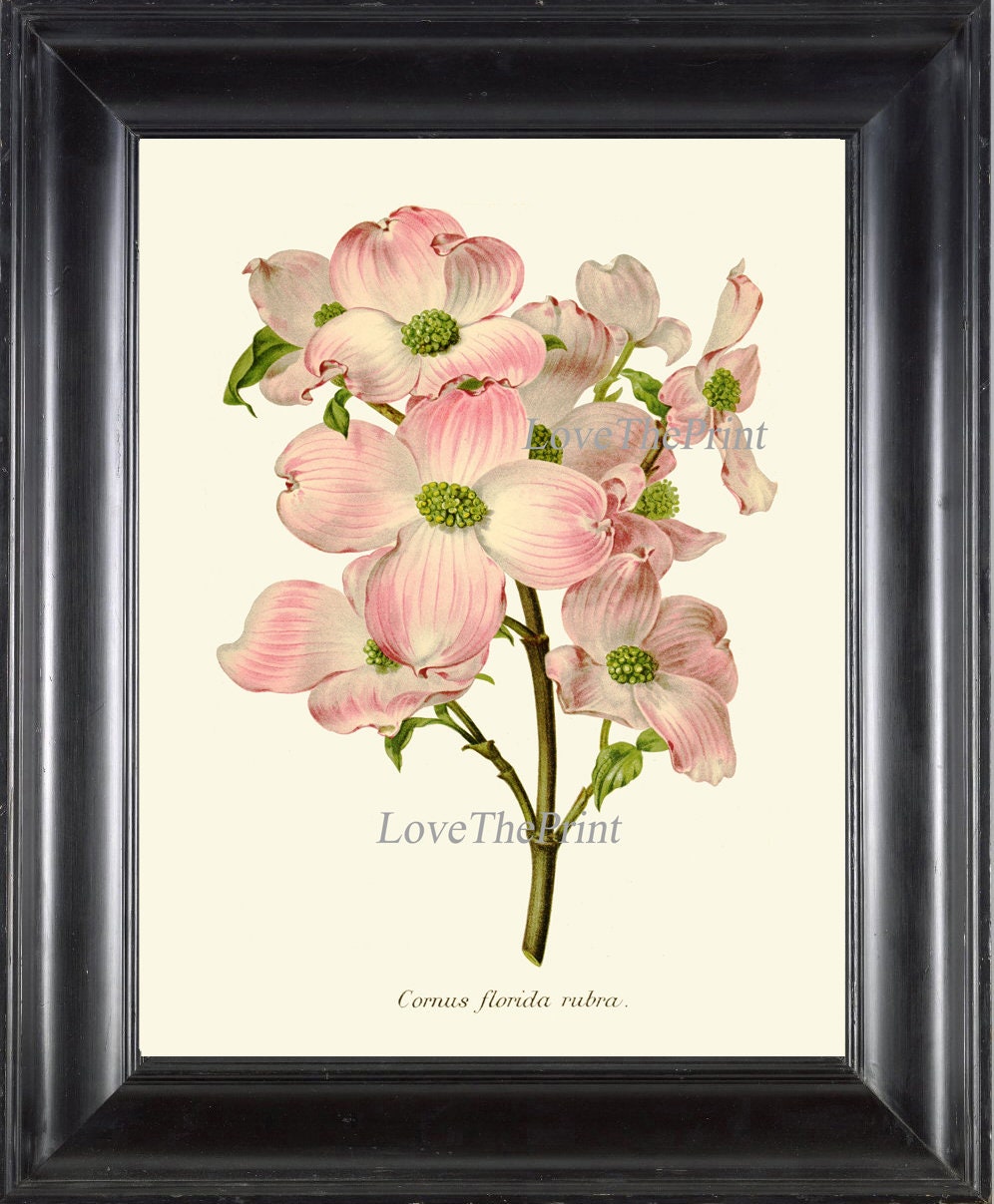The image depicts a detailed illustration of a Cornus florida rubra flower, framed in a thick wooden frame. The flower, with pink and white petals accented by green speckles in the center, is centrally positioned against a pristine white background. The stem exhibits shades of green and brown, adding to the botanical authenticity. Notably, the text "Cornus florida rubra" is inscribed at the bottom of the illustration, denoting the Latin name of the plant, while the phrase "Love the Print" appears twice, subtly watermarking the corners. The setting suggests a clean and minimalist style, emphasizing the flower's delicate beauty. The color palette includes touches of gray, tan, black, pink, white, yellow, and green, offering a harmonious visual experience.